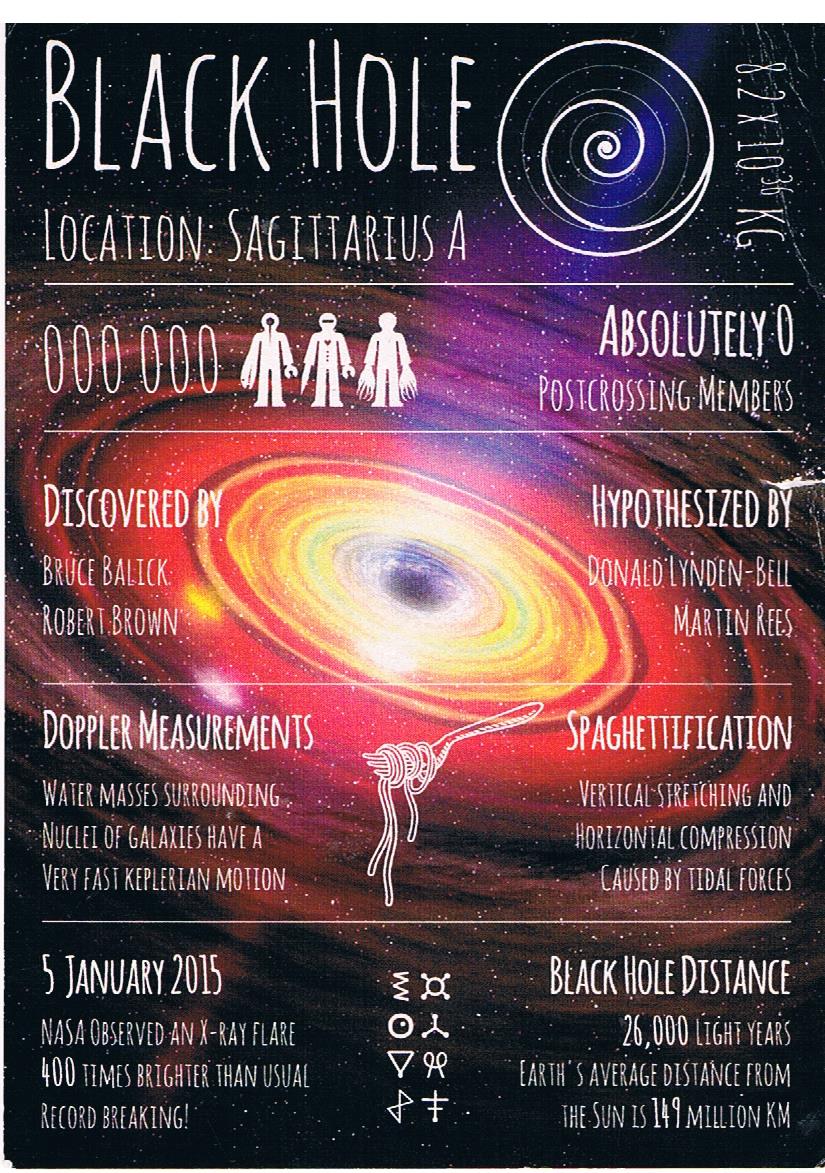The image depicts a vividly colored poster with a cosmic background resembling the Milky Way, filled with swirls of orange, yellow, and red, set against a star-studded sky. At the top, the headline reads "Black Hole," followed by the designation "Location: Sagittarius A" in prominent text. Below, three sketched alien figures are labeled "Absolutely Zero Post-Crossing Members."

Central to the poster, the contributions to the black hole's discovery and hypothesis are noted: "Discovered by Bruce Balick and Robert Brown" on the left, and "Hypothesized by Donald Lynden-Bell and Martin Rees" on the right. Further down, an illustration of a fork intertwined with a noodle is split into two sections: "Doppler measurements" on the left and "Spaghettification" on the right. 

Additional scientific details are included, such as "water masses surrounding," "nuclei of galaxies have a very fast Keplerian motion," and explanations of spaghettification involving "vertical stretching and horizontal compression caused by tidal forces." A significant date, "5th January 2015," marks NASA's observation of an X-ray flare "400 times brighter than usual," described as "record-breaking!"

At the bottom of the poster, alien symbols are intricately detailed, and in the bottom right corner, "Black Hole Distance: 26,000 light years" is stated, along with a comparative note: "Earth's average distance from the sun is 149 million KM."